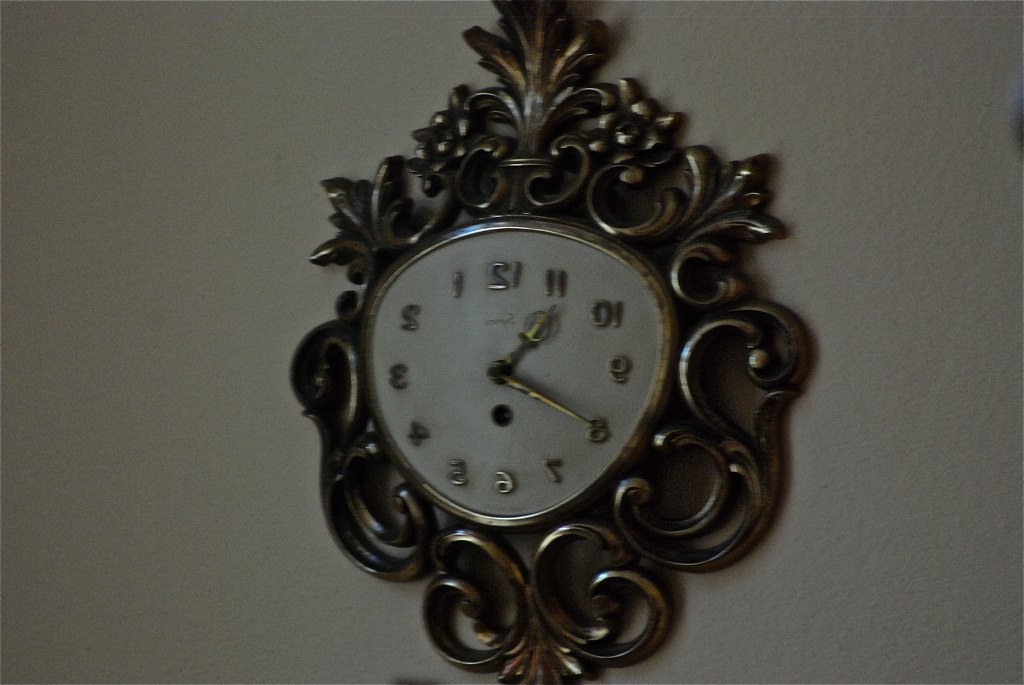This image depicts a metal wall clock set against a white wall, designed in an antique, Victorian style with a brass lacework frame that resembles a tropical, ornate sculpture. The frame intricately showcases patterns akin to tropical plants, feathers, and even leaf-like motifs, all rendered in a worn, patinaed, goldish-brass color, giving it a vintage charm. The clock face itself is white, featuring backward numbers in a mirrored arrangement, making it appear as though it runs counterclockwise. The 12 is reflected with the 1 on the left and the 2 on the right, and so forth, creating a unique visual effect. The hour and minute hands, which are also made of a tarnished gold metal, feature detailed designs, including a stylized king's crown motif on the hour hand, and rest between the 10 and 11 and on the 8, respectively. Below the hands, there is a small black dot, indicative of a wind-up mechanism beneath, further emphasizing its antique nature.